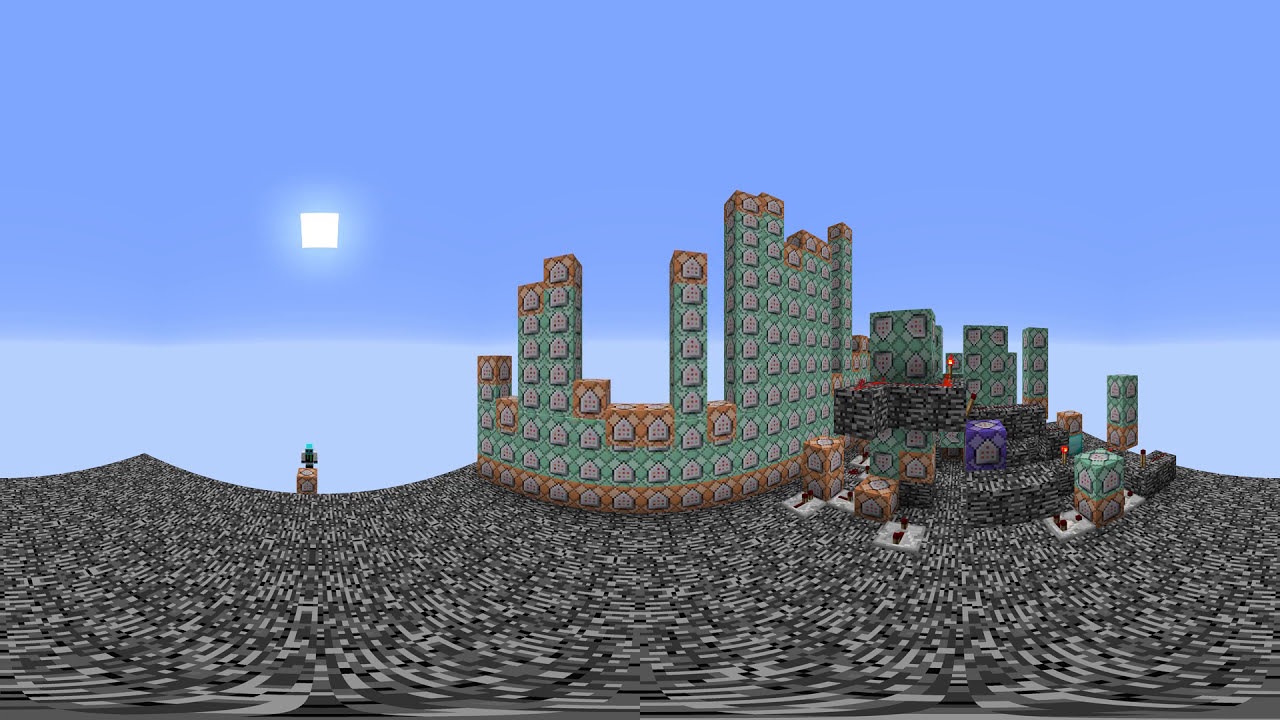The image appears to be a screenshot from the popular game Roblox, showcasing a vivid scene under a pale blue sky dominated by a blocky yellow sun. The ground is constructed from dark grey and black pixelated blocks, giving the impression of a textured surface. A cityscape of alternating green and orange blocks, each adorned with a house icon featuring white structures with orange windows, stretches across the scene. To the left, a character in a green outfit stands atop an orange housing block. The scene also includes a lit torch towards the rear, adding a touch of illumination. No text is present, creating a pure visual focus on the game elements, and the image conjures an outdoor environment despite being a video game setting.